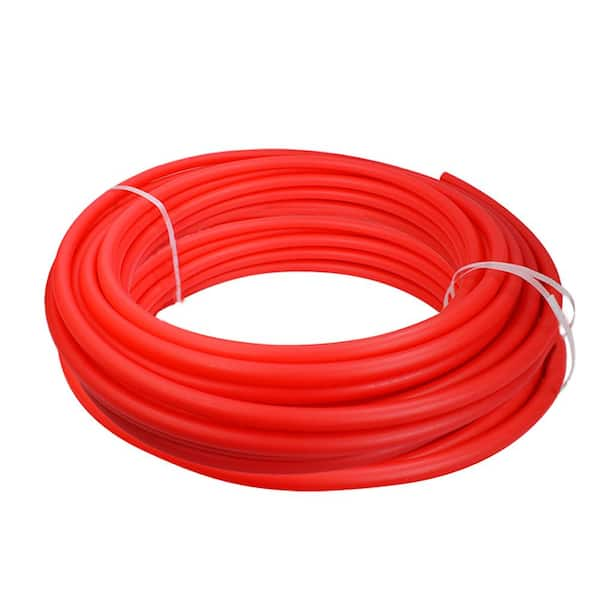This is a detailed photograph of a long, red hose, coiled neatly in a circular loop. The vibrant, striking red color of the hose is almost effervescent, making it highly visible against the completely white, context-free background. The hose is held together by two white plastic bands, one on each side. The band on the left side is more tightly secured, maintaining the hose's circular shape, while the band on the right side appears looser, allowing a slight expansion of the coil. The hose does not have any nozzle or connector. The shiny, smooth surface suggests a high-quality material, possibly designed for irrigation or plumbing purposes. The image's professional quality hints that it might be intended for a hardware store advertisement.